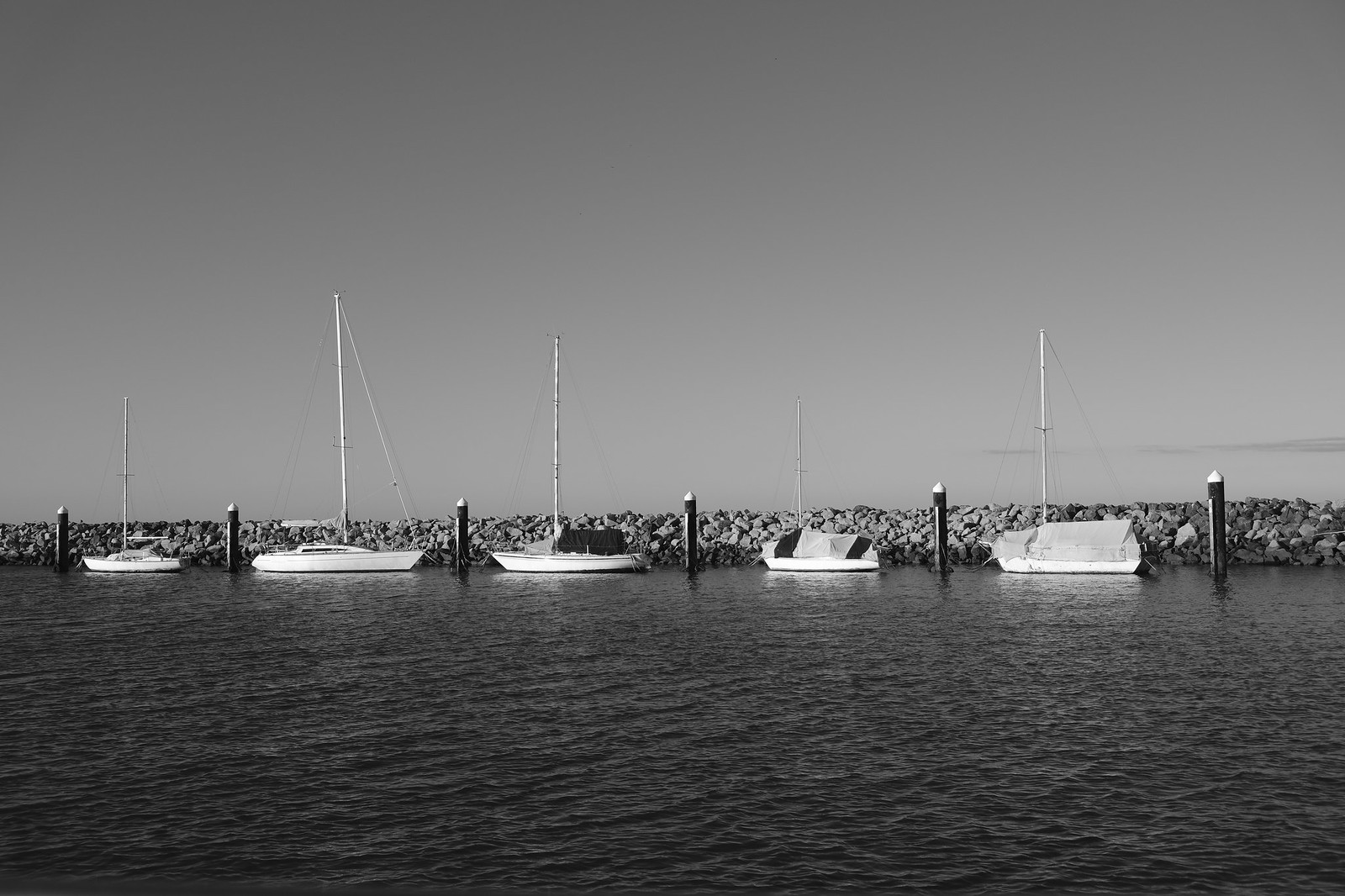This black and white photograph captures a tranquil scene of five sailboats anchored along a rugged seawall made of large gray rocks. The sailboats vary in size and are aligned horizontally from left to right. None of the boats have their sails up. The first sailboat on the left is small and white, followed by a slightly larger one with the tallest mast. The third sailboat has a smaller mast and features a black covering. The fourth boat, even smaller, also has a black and gray tarp, while the fifth boat has a mast taller than the fourth, but shorter than the second. Black mooring posts are placed between each sailboat, offering potential tie-off points. The foreground reveals calm ocean or lake water, adding to the serene atmosphere. In the background, the sky is mostly clear with a hint of a cloud in the lower right center, enhancing the peacefulness of this protected bay or dockside area.